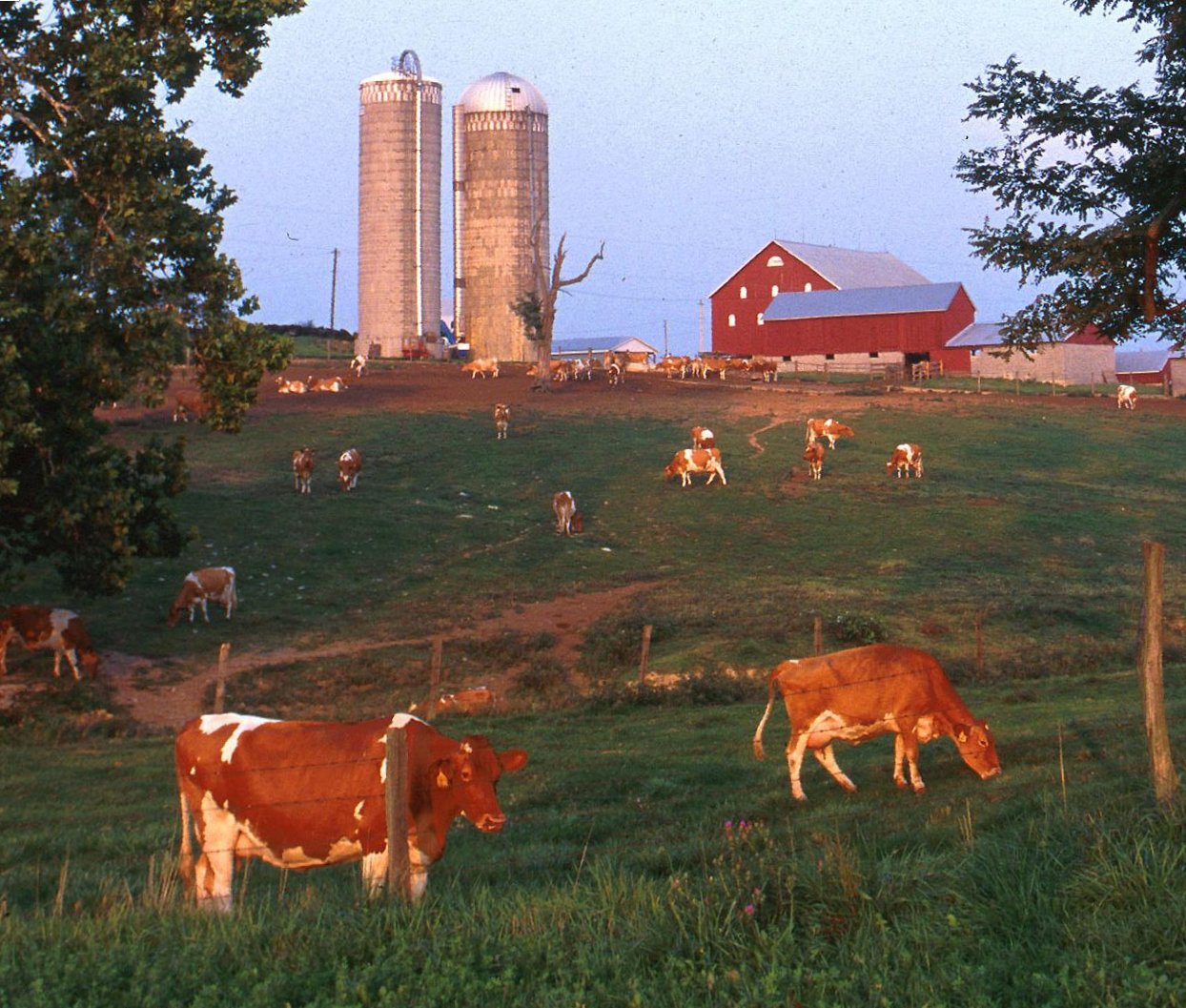The image depicts a serene farm scene featuring a lush, green field dotted with numerous cows. The cows, a mix of white and orange colors, are scattered across the expansive grassland, which is interspersed with narrow dirt trails. In the background stands a large, reddish-brown barn, flanked by two substantial gray silos. A barbed wire fence in the foreground encloses the field, keeping the cows within its bounds. To the left and right edges of the scene are two verdant green trees, adding to the pastoral charm. Further in the distance, a row of electrical poles with horizontal wires stretches towards the horizon. The sky above is a clear, light blue, devoid of any clouds, creating a tranquil and picturesque atmosphere.